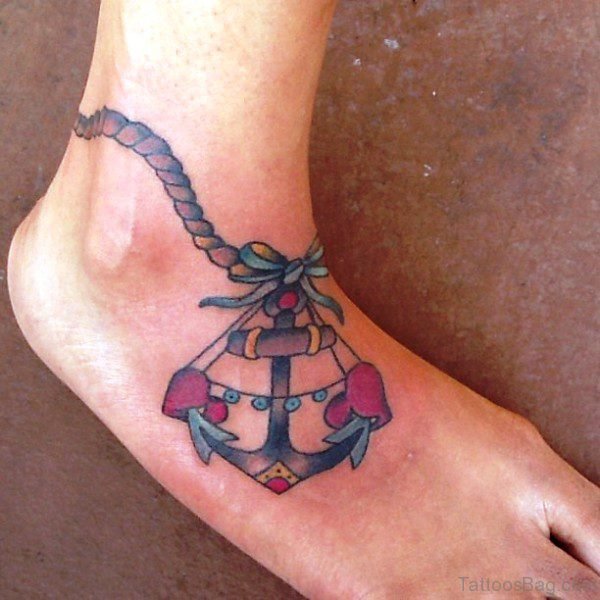This image captures a close-up photograph of a person's foot, prominently featuring an ankle tattoo. The focal point of the image is the tattoo itself, which artistically wraps around the ankle with a rope-like design that leads to a bow and a stylized anchor. The anchor, decorated with green ribbons and red hearts, gives a detailed and intricate look. The foot is placed against a marbled, brownish background that resembles skin or an odd, almost fish-scale-like surface, which contributes to the unusual and stark appearance of the scene. The tone of the foot is notably reddish, and some proportions appear somewhat distorted, adding to the overall impression of the image. Additionally, there is a subtle watermark in the lower right corner of the image with the text "tattoosbag.com," suggesting the photo may have been sourced from the internet. The color palette of the picture includes shades of brown, tan, olive, red, light blue, black, gray, and yellow, primarily centering on the foot but slightly off-alignment to the left. The setting hints at a personal environment such as a home or possibly a tattoo shop where the tattoo has just been freshly done.